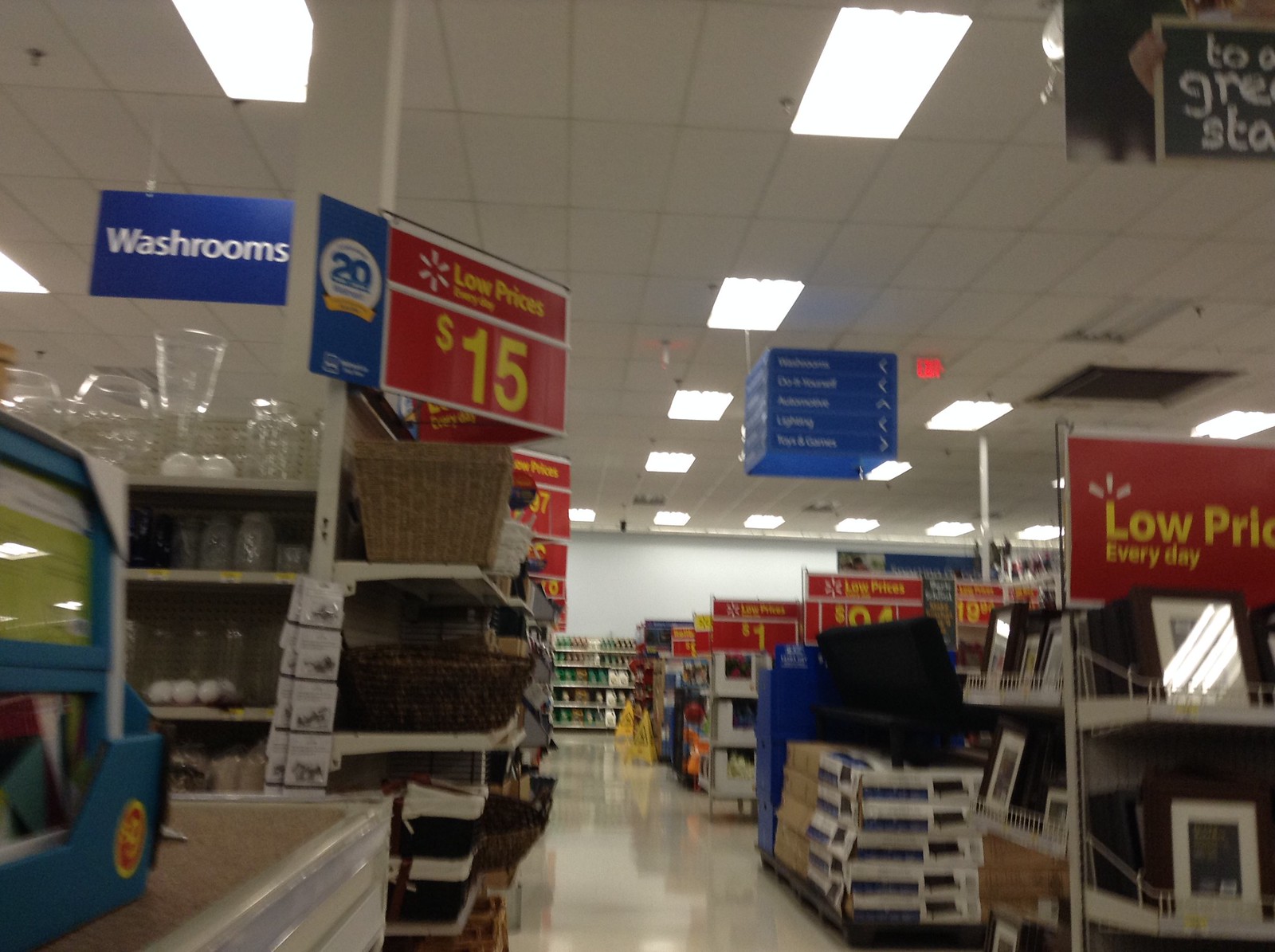The image appears to depict a Walmart store interior. Dominated by blue signage, the left side features a prominent blue sign that reads "Washrooms," adjacent to another large blue sign declaring "Low Prices" accompanied by a small star symbol. Below this sign, there is a basket, indicating the store's basket section. Additional red signs scattered throughout the scene emphasize "Low Prices Every Day." A square, blue directory with white text is also visible, helping customers navigate the store. Bright overhead lights illuminate the entire space. On the right-hand side, there is a display of picture frames. The overall atmosphere, color scheme, and signage strongly suggest the store is indeed a Walmart.